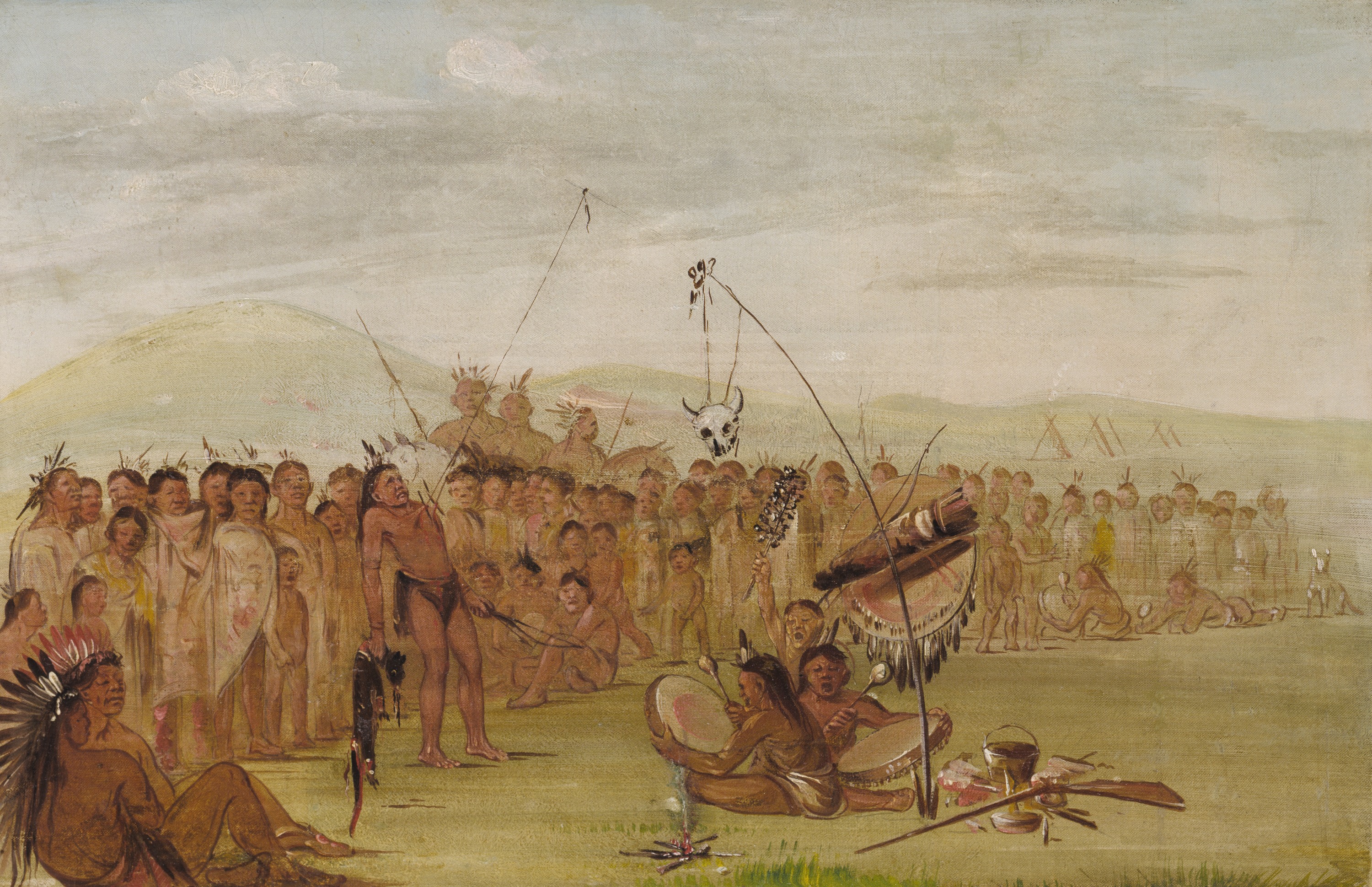The painting depicts an outdoor ceremony involving Native Americans, where a large group of men, women, and children with brown skin tones have gathered. Many are minimally clothed or naked, wearing traditional headgear and shawls. The focal point of the scene is a man connected to a fishing rod-like torture device that hooks into his chest, forcing him to bend backward while holding a dead animal in his right hand. The ground is grassy, and two other Native Americans are seated, rhythmically beating drums. A skull is hanging from the intricate apparatus used in the ceremony. In the background, small hills and teepees are visible under a blue sky with dark clouds. The atmosphere is vividly captured, evoking a sense of ritualistic intensity and communal involvement.